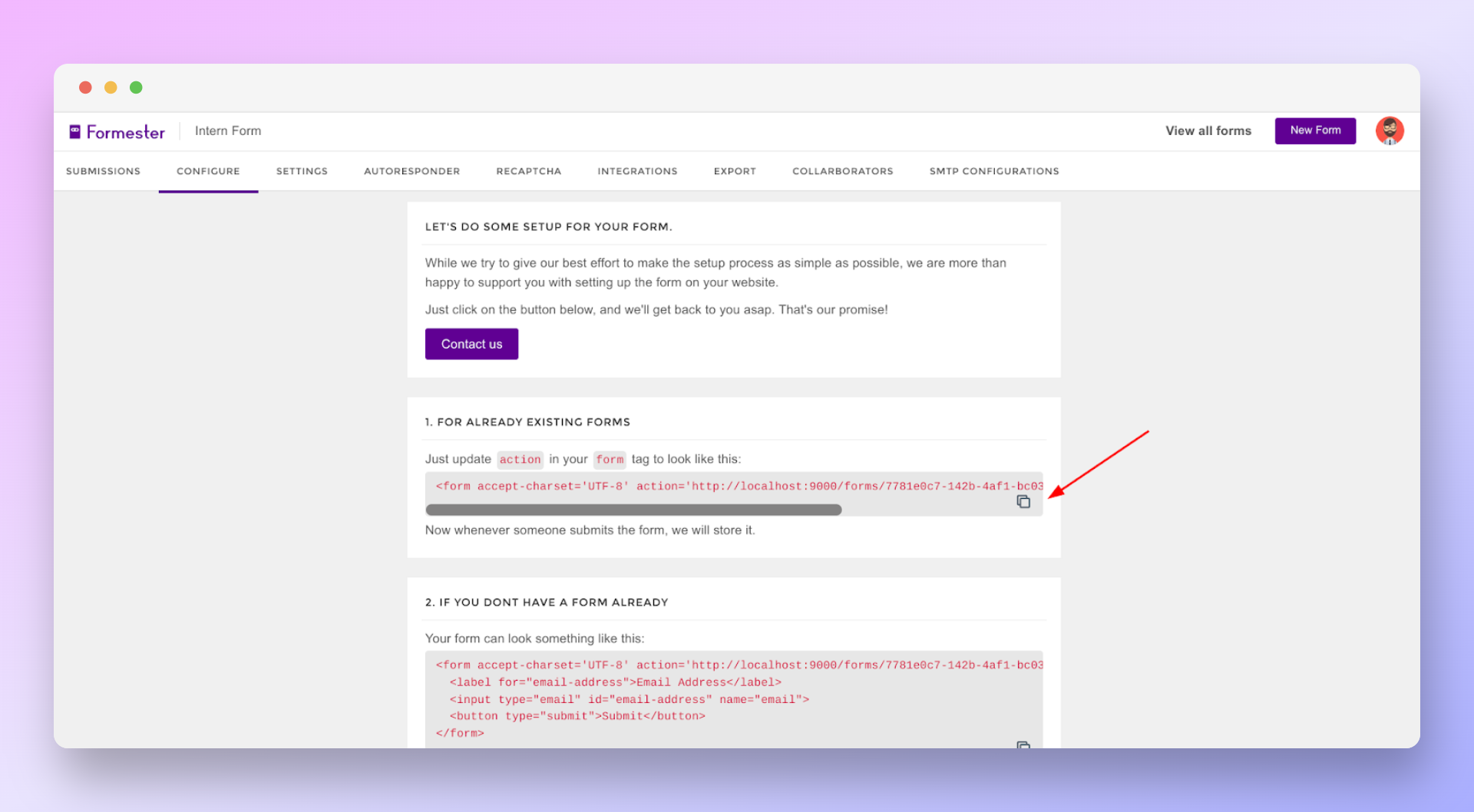The image depicts a web page encased in a lilac and purple border. The main section of the web page features an off-white background. In the upper left corner, there are three small dots in red, yellow, and green. Directly below these dots, the word "Foremaster" is prominently displayed in purple text. To the immediate right of "Foremaster," there is smaller black text reading "intern form."

Beneath the menu options, the text "Let's do some setup for your form" is visible. Additionally, there is a purple button located further down the page, which bears the text "Contact Us" in faint white lettering. The rest of the space is taken up by the form content.